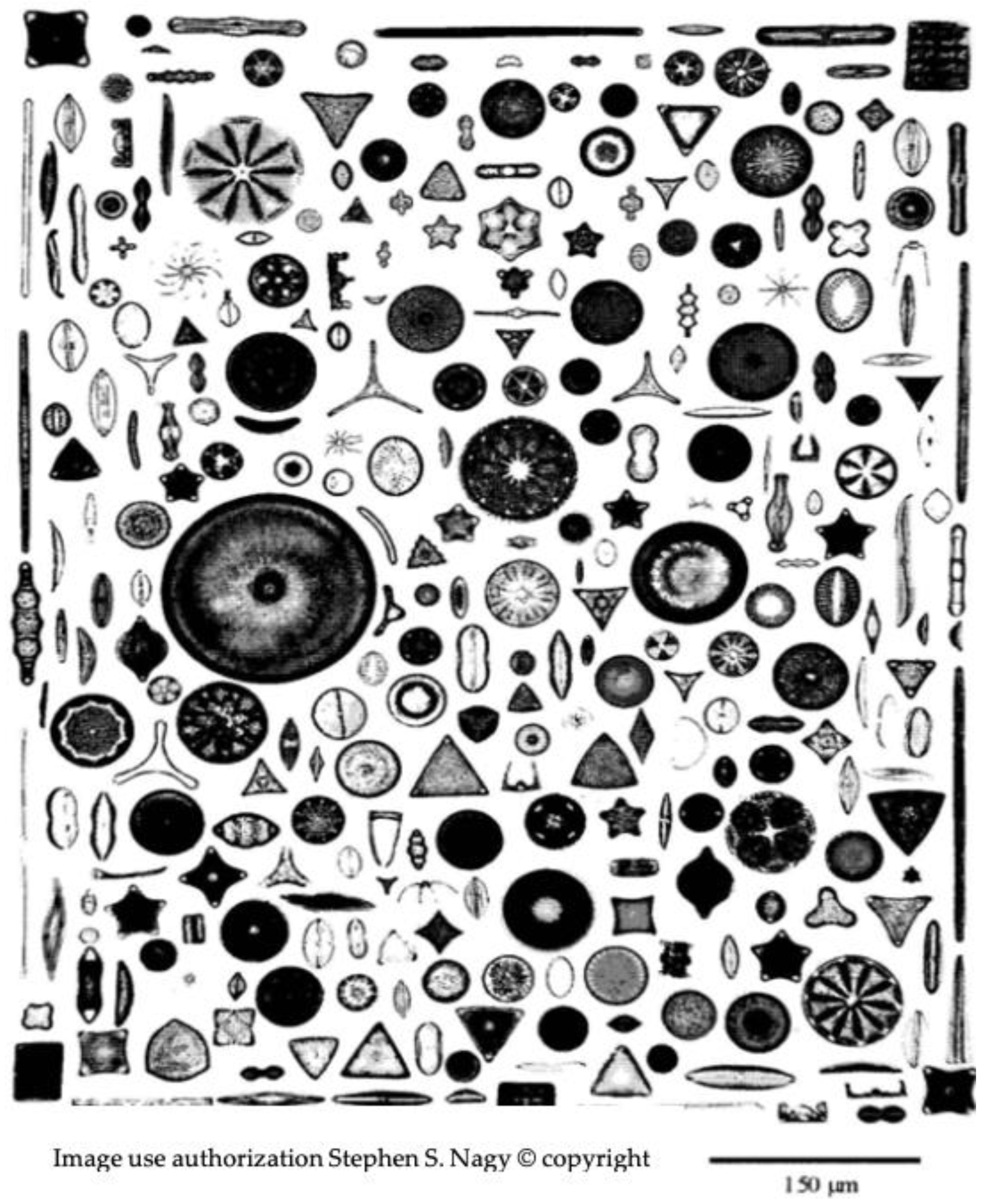The black and white image is a detailed rectangular graphic featuring a diverse array of geometric shapes, including circles, triangles, ovals, and more abstract forms such as boomerang-like shapes and leaf-like patterns. These shapes vary in size and design, with some featuring distinctive inner patterns like a spinning wheel. The background is white, and the graphic is bordered with four squares at each corner. While some shapes, especially circles and triangles (including upside-down ones), are more frequent, each shape appears to have unique attributes, with many circles having holes in them. There seem to be around a hundred designs spread throughout the image. The lower part of the graphic includes a watermark that reads "Image Use Authorization Stephen S. Nagy Copyright," and there's a note labeled "150 mm," potentially indicating the size. The image resembles wrapping paper, a magazine illustration, or could serve as a brain teaser or coloring activity, allowing for a creative outlet.